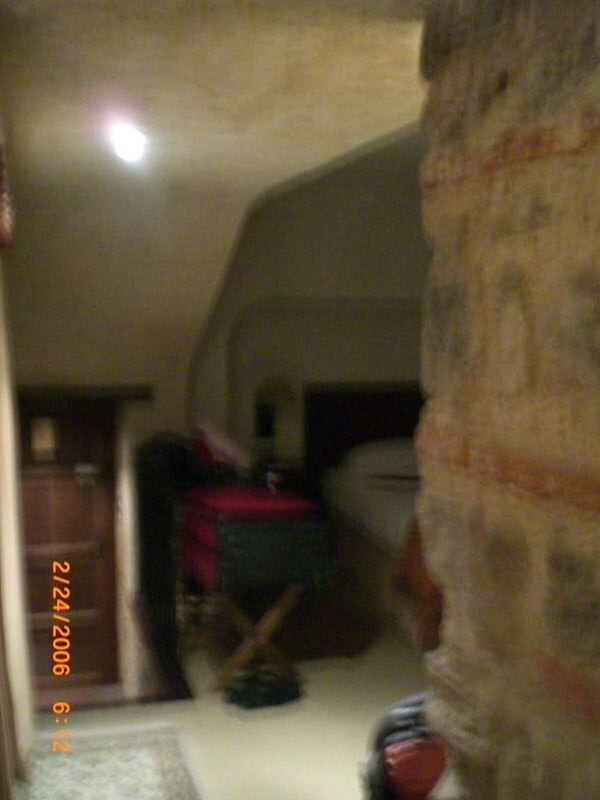This image depicts an attic or top-floor room in a house. On the left side of the frame, turned on its end, is a clear marking that reads "224-2006 at 612." Dominating the right side of the image is a large brick structure resembling a chimney. The room contains various furnishings including an unmade bed, where the pillow, sheet, and quilt are visibly disarrayed. Adjacent to the bed, there is a dresser. A small, folded wooden stool sits next to the bed, topped with a case that is gray on the ends and red in the center and top, akin to a suitcase. Despite the blurry quality of the photo, the detailed elements of this attic room create a vivid sense of the setting.